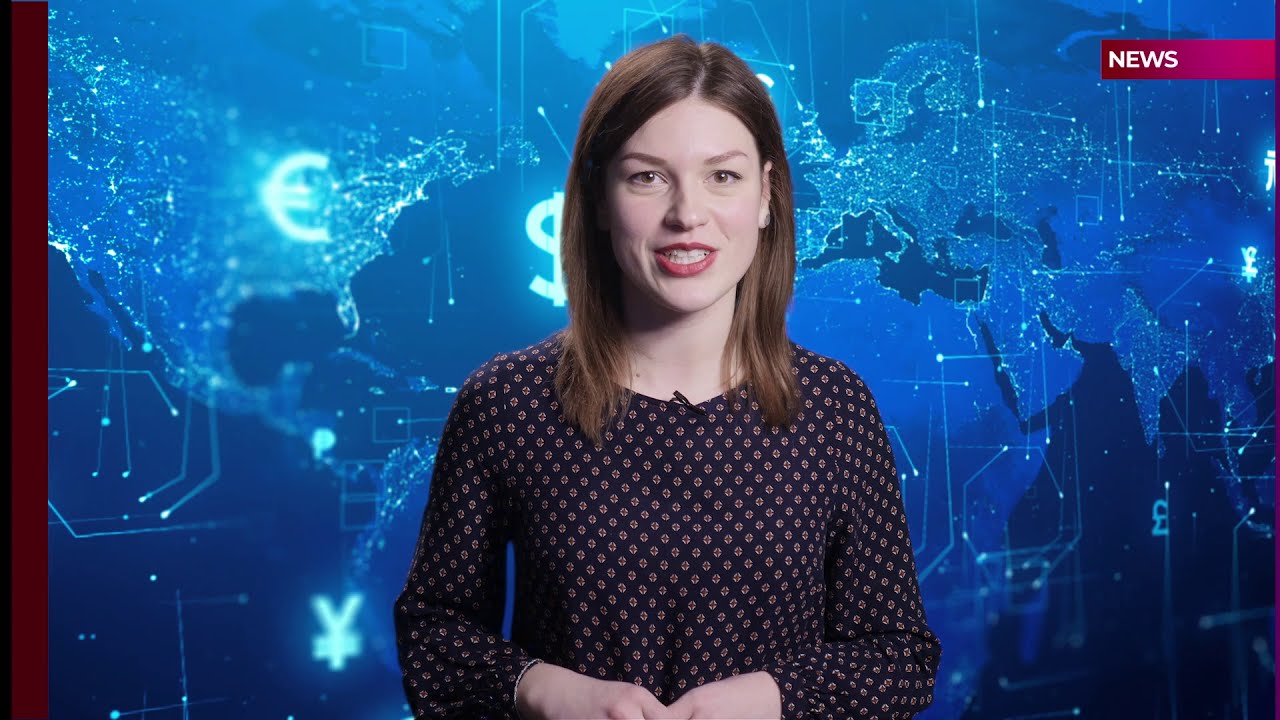The image depicts a still from a news broadcast featuring a white female anchor with shoulder-length brunette hair. She has red lipstick applied and is positioned with her mouth slightly open, as if she is about to speak. She is wearing a navy blue long-sleeve shirt adorned with a small dot pattern, and a clip-on microphone is attached to the top of her shirt. Her hands are clasped together in front of her as she faces forward. The background features a blue world map with various currency symbols including the dollar, yen, euro, and pound signs. In the top right corner of the image, there is a red rectangle with the word "NEWS" in bold white capital letters. The setting is indicative of an imminent news presentation, suggesting the anchor is preparing to delve into a globally relevant subject.